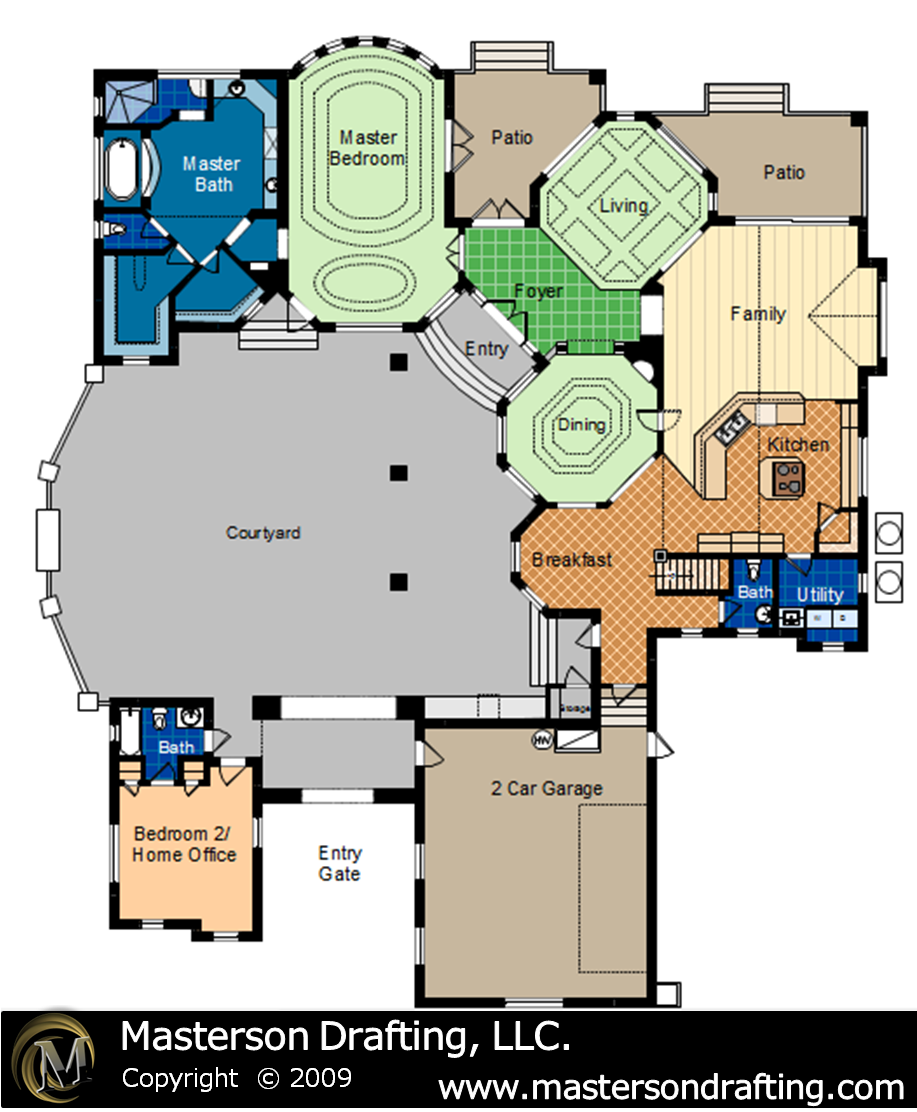Blueprint of a residential home designed by Masterson Drafting LLC (© 2009, www.mastersondrafting.com). The layout includes a two-car garage and several living spaces designed for flexibility and comfort. Adjacent to the garage is Bedroom 2, which can also function as a home office, complete with an ensuite small bathroom. Behind this room lies a serene courtyard leading to the main entryway. 

Inside, a breakfast nook seamlessly transitions into a modern kitchen, complemented by a dedicated dining area. The family room opens to a cozy patio, perfect for outdoor entertainment. Additional living space includes a separate living room that leads to a secondary patio. The master suite comprises a spacious bedroom and an elegant bathroom featuring a large tub. The blueprint captures a thoughtful design aimed at maximizing both indoor and outdoor living experiences.